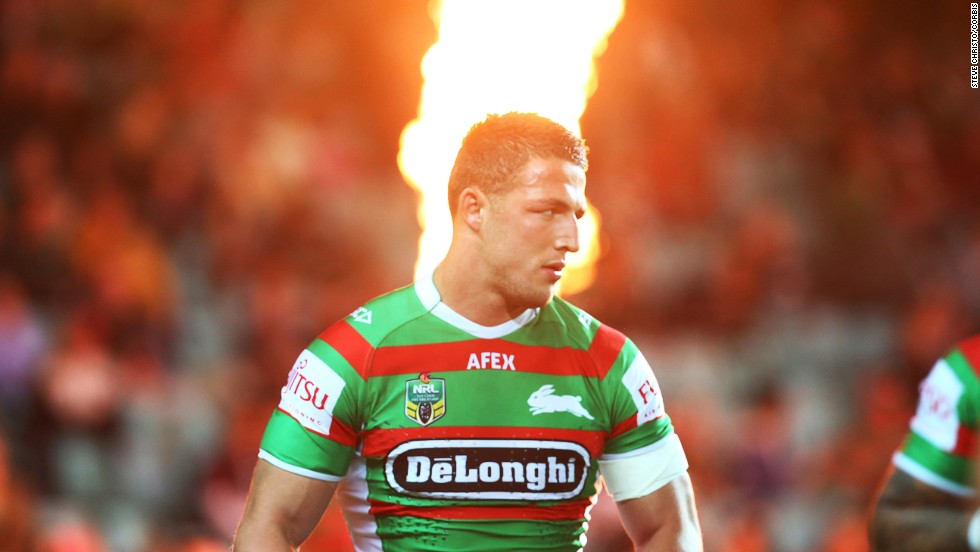The image features a Caucasian man, characterized by his medium-brown, short hair and a prominent, slightly pointy nose. He is captured from the front and right side, showcasing his muscular build and wearing a vibrant green sports shirt. This shirt prominently features a thick red stripe that extends over the shoulders and chest, framing the bold, white text "APEX" across the center. On his left chest, there's a white rabbit emblem, while on the right chest, inside a small yellow box, the letters "NRL" are vaguely visible. Each upper arm bears a white box with red letters, though the text is not entirely legible. Beneath the rabbit emblem is another red stripe, followed by a black box outlined in white, inscribed with the word "DELONGHI." Another red stripe runs below this box, completing the shirt's design with the remaining green fabric.

In the background, what appears to be flames give the illusion of pouring out from the man's shirt, though it is actually a visual trick created by the scenery. The backdrop includes a sea of people, possibly seated in rafters, creating a bustling atmosphere. The crowd is dotted with orange hues, adding to the vibrant and dynamic feeling of the scene. Another individual wearing the same sports shirt is partially visible on the right side of the frame. The overall composition of the image, combined with the illusionary flames and crowd, captures a moment full of energy and excitement.